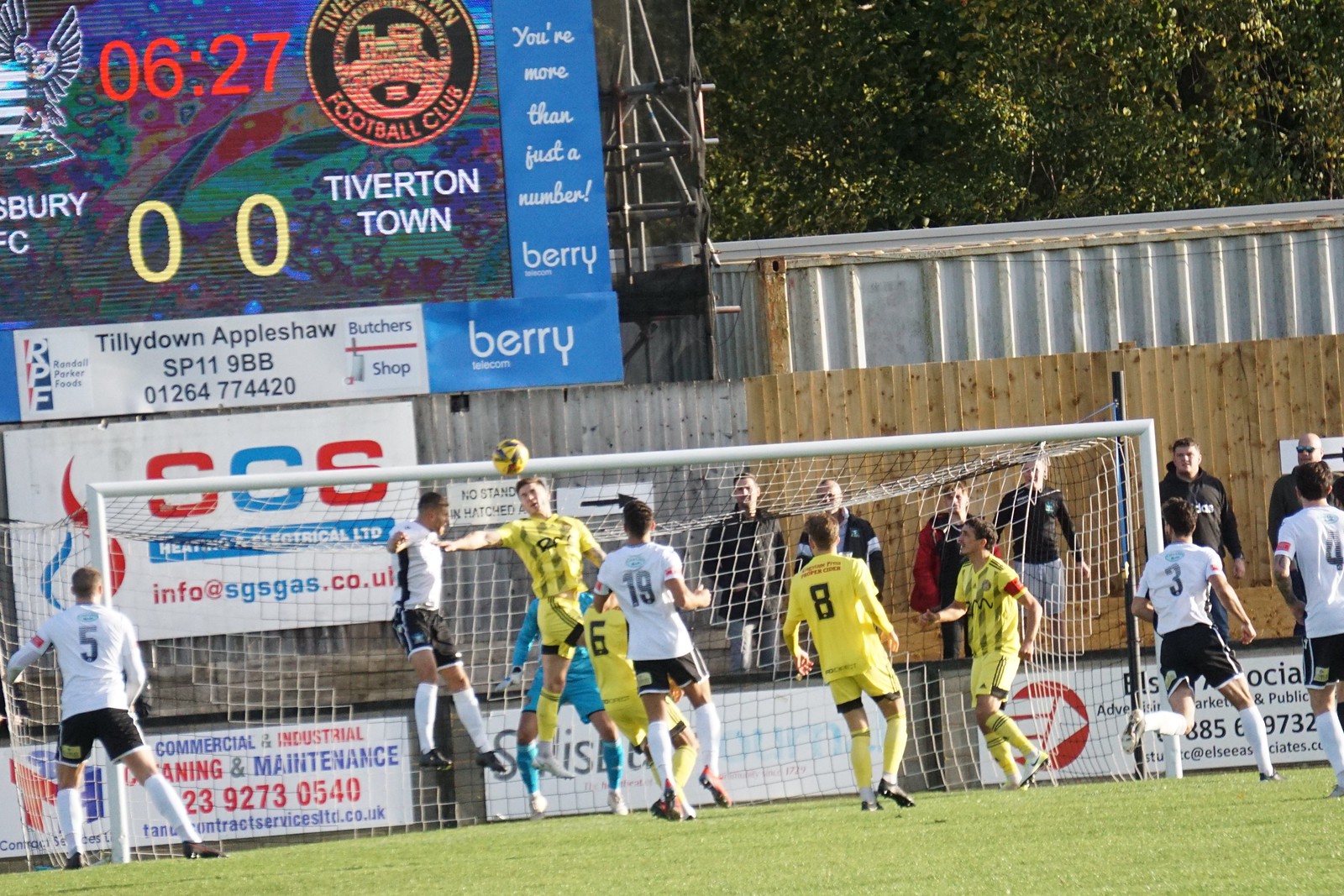The photograph captures an outdoor soccer game in progress, viewed towards a goal where both teams have clustered. The scene is intense with players in white jerseys with black shorts and yellow jerseys with yellow shorts converging on a yellow ball. Two players, one in yellow and the other in a different kit, are mid-air, competing for a header. The yellow-dressed player appears to be the goalkeeper, making a crucial play. Behind the players, a netted goal with a white railing stands prominent, and a line of what seems to be coaches and staff are visible. In the background, above a metal wall and awning, a scoreboard displays 6:27 minutes remaining and a score of 0-0. The scoreboard, which includes a blue border with sponsorship advertisements, highlights Tiverton Town’s team crest—a circular emblem featuring a castle. Additional background details include a shed, foliage, and various other sponsor signs, all under the bright daylight providing natural illumination to the dynamic scene.